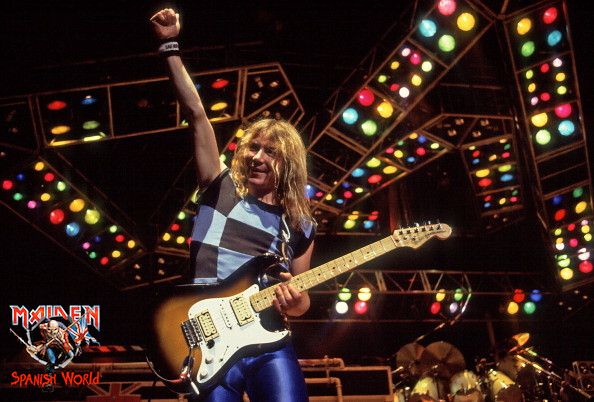The image captures an indoor concert scene featuring a central male performer with long, wavy blonde hair parted in the middle. He is energetically posing with his right arm lifted, making a fist, and smiling while looking to his side. He is dressed in a blue and black checkered sleeveless top paired with shiny blue pants. In his left hand, he holds a two-tone electric guitar, brown at the bottom and lighter towards the middle. The vibrant background is a striking display of multicolored lights including red, yellow, green, blue, and white, scattered across the ceiling. Behind him on stage, a drum set is visible. Notably, on the left side of the image, the word "Maiden" is written in red, accompanied by a menacing skull with a British flag, and at the bottom, "Spanish World" is inscribed in similarly haunting red letters.